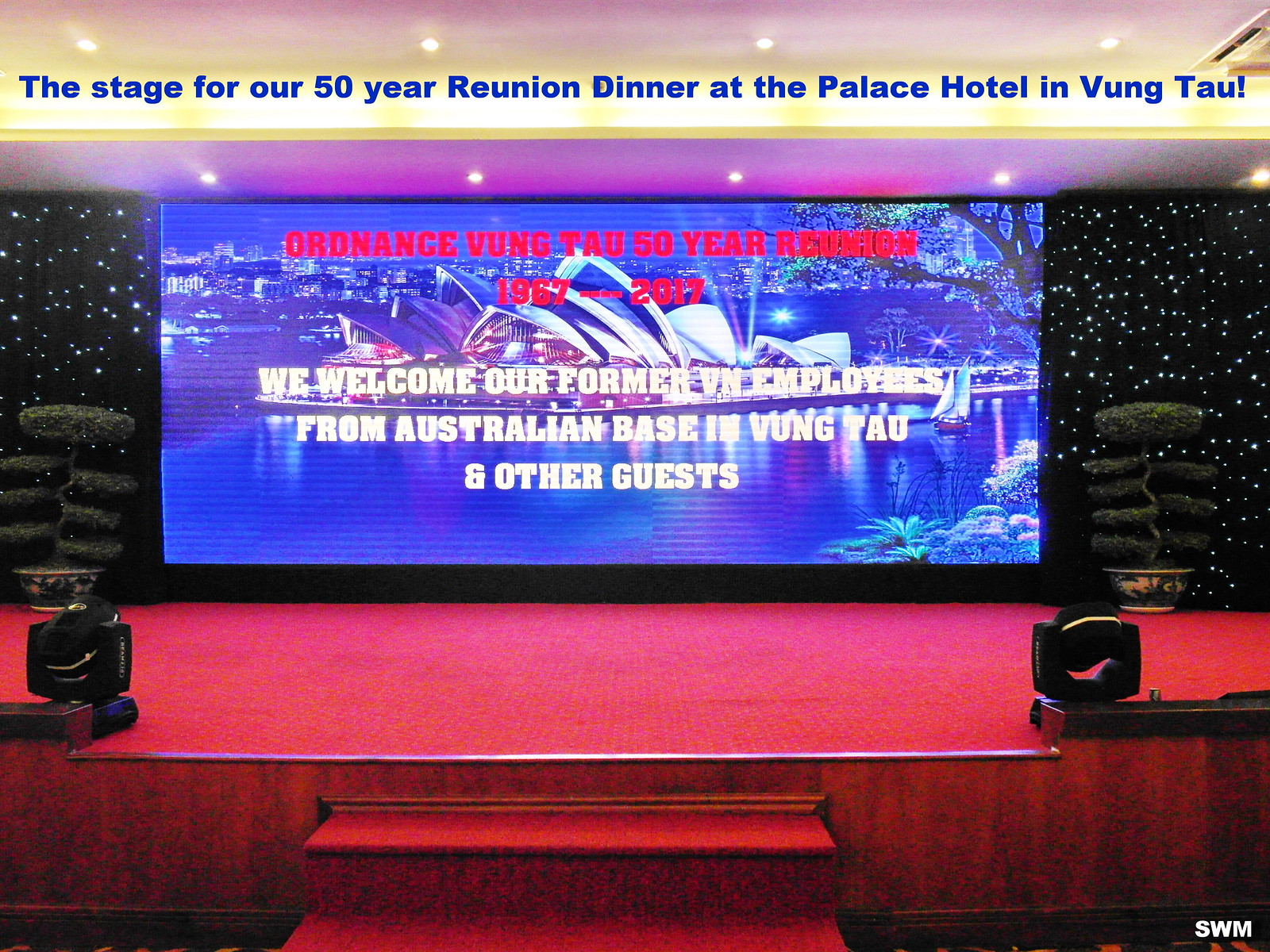This photograph showcases a grand stage adorned in red carpets, situated at the Palace Hotel in Vung Tau for the Ordinance Vung Tau 50-Year Reunion dinner (1967-2017). The stage features a red carpeted staircase leading up to it and two black speakers positioned at the front. A prominent feature is the large screen or banner in the backdrop, which reads, "Ordinance Vung Tau 50-Year Reunion 1967-2017. We welcome our former VN employees from Australian base in Vung Tau and other guests," with an image of the Sydney Opera House over water in the background. Flanking the screen are two tall plants in round planters. Additionally, the black curtain behind the screen adds a touch of sparkle and glitter. At the top, another banner declares, "The stage for our 50-year reunion dinner at the Palace Hotel in Vung Tau." The stage setup includes lighting at both corners, creating a vibrant and welcoming atmosphere for the celebratory event.